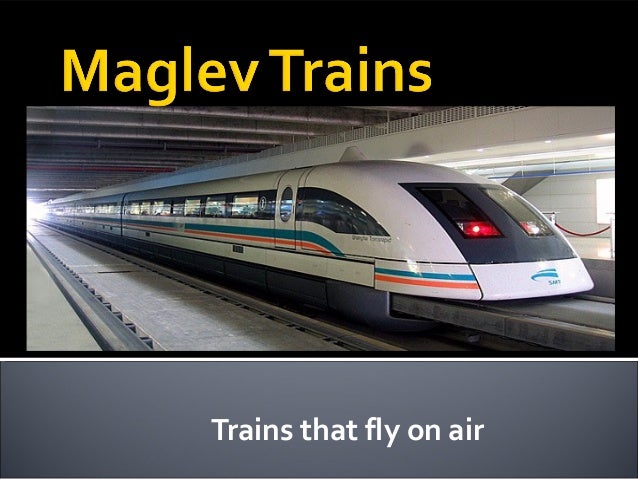This image showcases a sleek, white Maglev train stationed on a platform. The front of the train tapers off like a bullet and features two windows and a blue logo below them. Distinctive blue and orange stripes decorate the train, running from the front to the back along its body. A large black border frames the picture, with the words "Maglev trains" in bold yellow lettering at the top and "trains that fly on air" in white lettering on a gray background at the bottom. The train appears to be still, yet its aerodynamic design and the glowing light in the background suggest the idea of speed and innovation. This captioned image might be part of a presentation or educational material, highlighting the advanced technology of Maglev trains, which operate without touching the track, giving the impression of floating and high-speed travel.